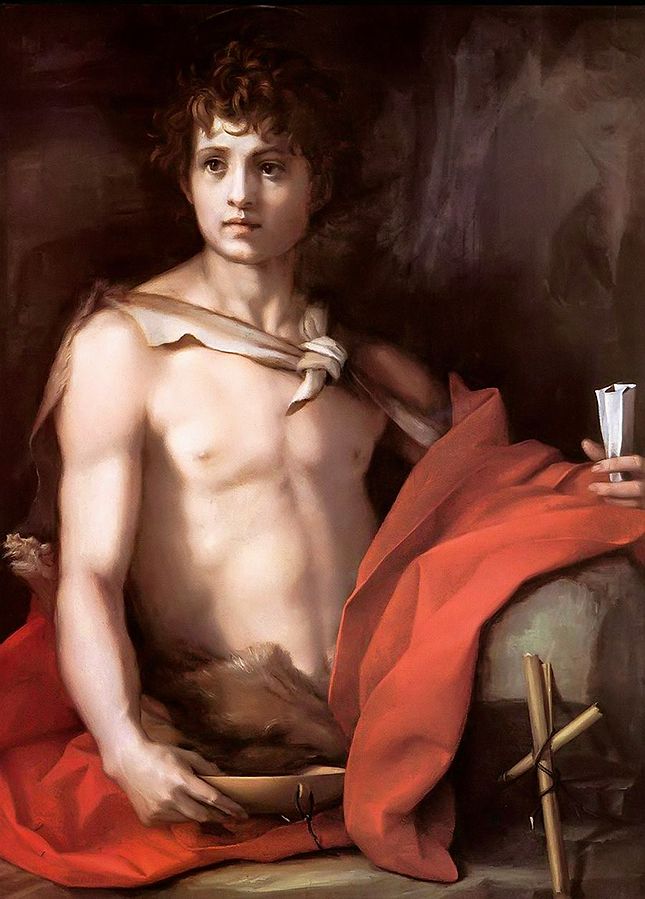This portrait artwork depicts a young, white-skinned man with brown, disheveled curly hair, sitting down with his legs not visible. He appears to be shirtless, revealing his lean, muscular chest and arms. Draped over his shoulder is a red cloth, resembling a cape, and another red cloth is wrapped around his waist area. The man is holding a bowl with a brown substance in his right hand and a silver drinking item in his left hand. His facial expression conveys innocence, and he gazes slightly to the left. The background features a dark brown, almost black wall with white marks and a small wooden cross on the lower right side, evoking a classical and somewhat historic atmosphere.